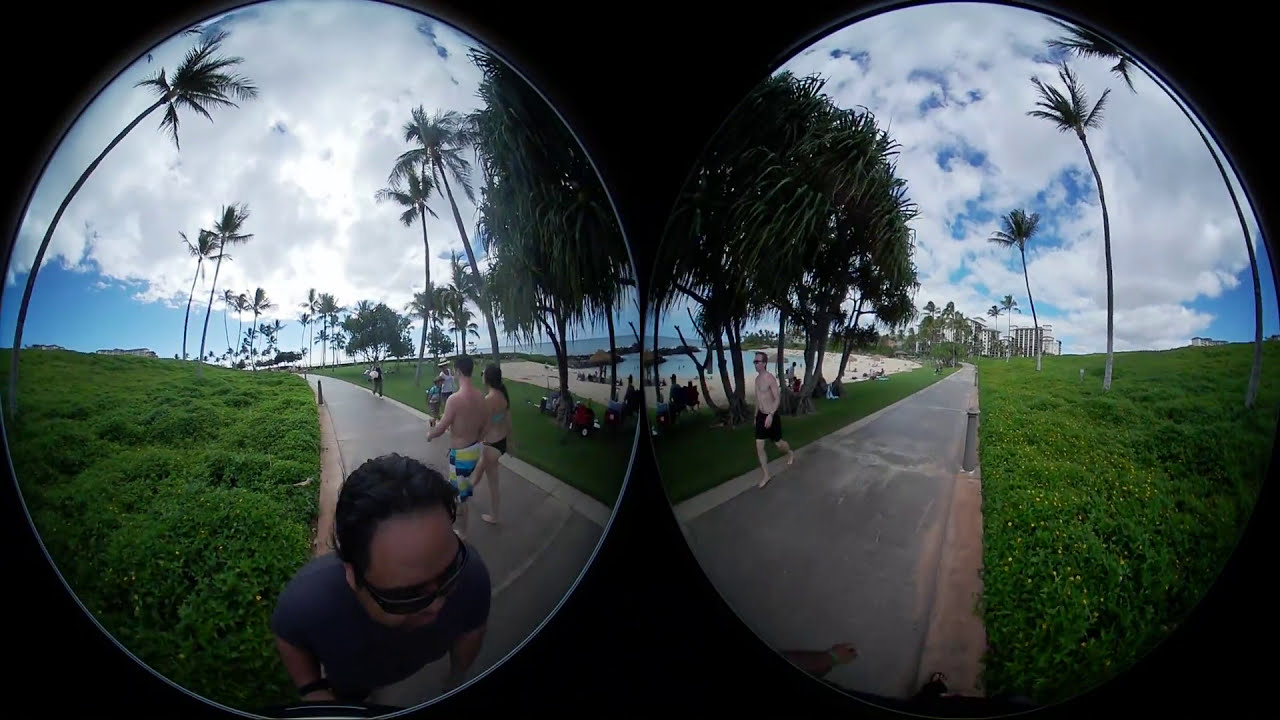The image presents a lively scene from a tropical beachside walkway captured using a 360-degree panoramic view, divided notably into two sections. The foreground features a concrete walkway bustling with people dressed in summer attire, including bathing suits, with some individuals barefoot, reveling in the warm, albeit slightly cloudy, daytime weather. Central to the image is a small bay dotted with relaxed beachgoers, set against a backdrop of ocean waves breaking on distant rocks. Midway, the scene transitions to people enjoying picnics on a grassy patch, surrounded by the shady comfort of palm trees. In the background, more palm trees tower over the landscape, enhancing the tropical ambiance. The panoramic shot includes two distinctive circular lenses that divide the photo. On the left side, partially obscured by shadows, a person appears at the bottom of the image, possibly the photographer, with their identity largely hidden. Meanwhile, two individuals in bathing suits walk away, further contributing to the laid-back beach atmosphere. The right section shows additional sandy areas, water, and more foliage, reinforcing the scenic and vibrant environment of this tropical locale.